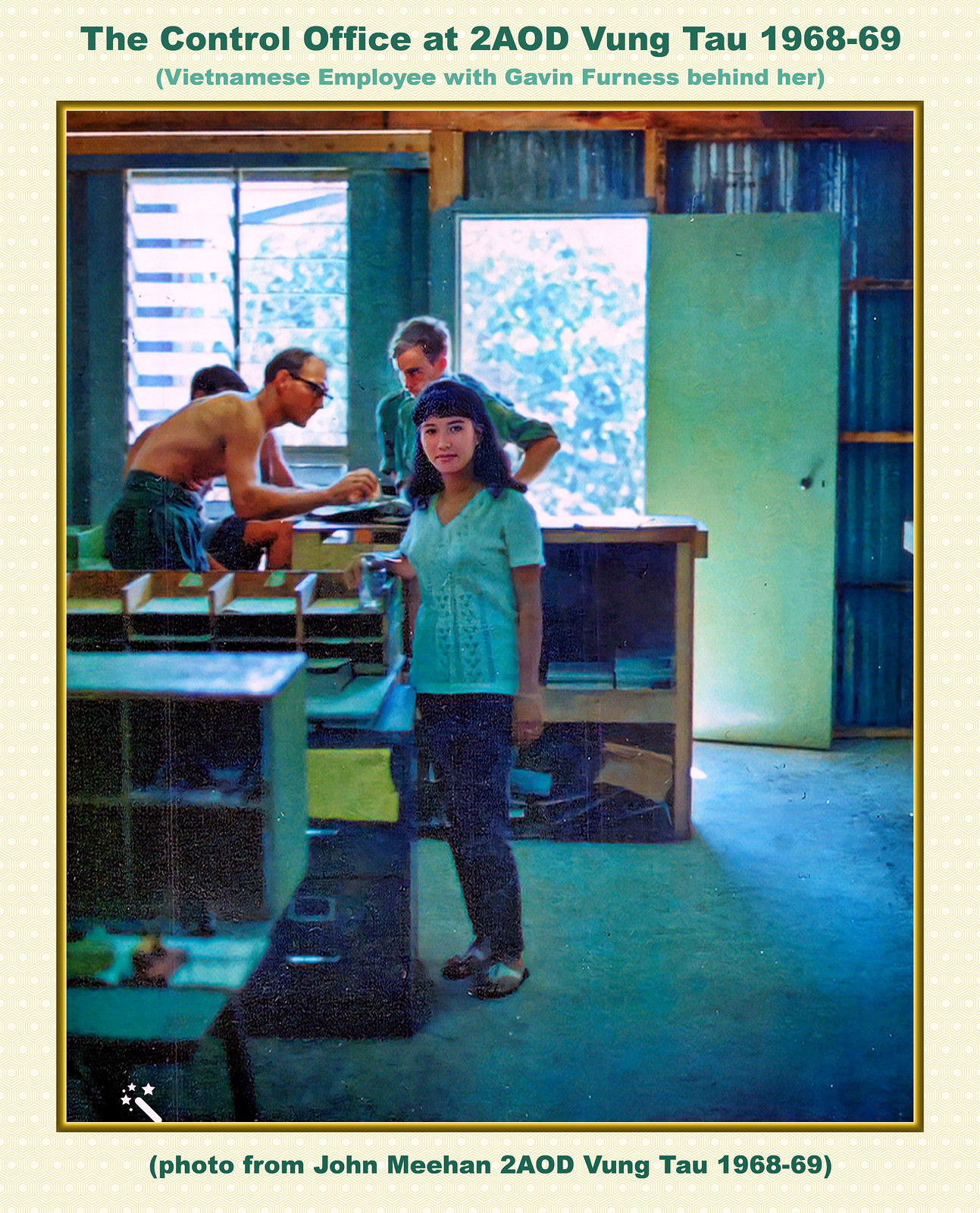This detailed image, appearing to be part of a pamphlet, features the control office at 2 AOD Vung Tau, Vietnam, during 1968-69. The overall background is light yellow, framing a photograph encased in a golden border. The scene captures a room with distinctive green floors, green tin walls, open glass windows, and an open green door leading outside, showing glimpses of trees and daylight. 

Inside, a young girl with shoulder-length black hair stands wearing a green half-sleeve top, blue jeans, and slippers. She gazes directly at the camera, smiling, with a hand resting on a piece of furniture. Several desks and cabinets cluttered with papers and files are arrayed to her left, while a significant desk and cabinet occupy the background.

A bare-bodied man, wearing glasses and black pants, is bent over the desk, writing, with another shirtless man seated behind him. Additionally, a man in a green shirt stands by, observing the scene. The photograph is captioned at the top with "The control office at 2 AOD Vung Tau 1968-69," and noted at the bottom as "photo from John Meehan, 2 AOD Vung Tau 1968-69."